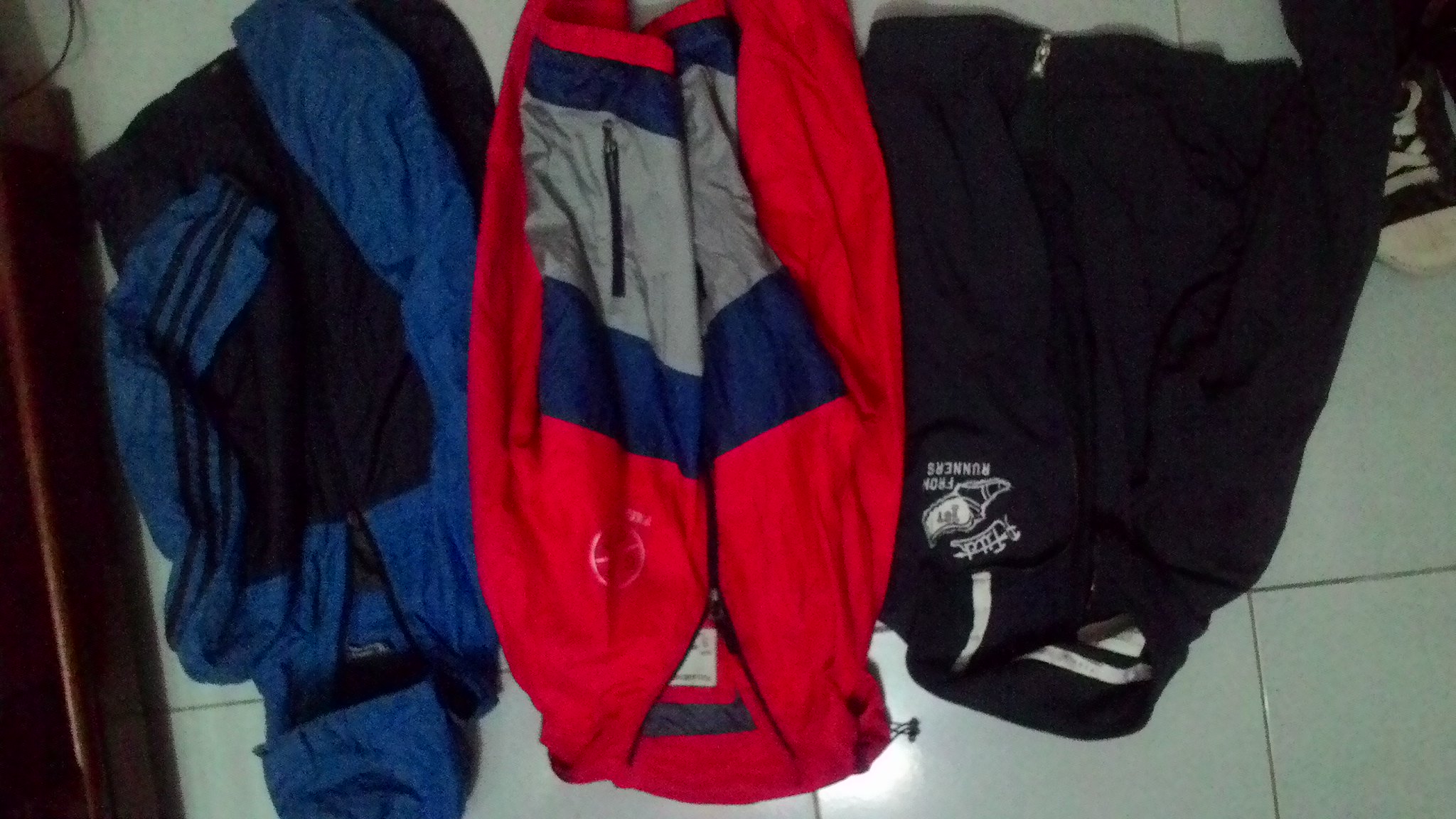This photograph showcases a collection of neatly folded sports jackets on a white tile floor. The jackets are arranged side by side, each with its own distinct design and color pattern. From left to right, the first jacket is predominantly blue with dark blue stripes and features a hood. Next to it is a red zip-up jacket with intricate blue and gray striping through the middle and a round white circle at the top. The final jacket is primarily black with white lettering that appears to say "FORM RUNNERS" along with an image of a foot, indicating an athletic theme. To the upper right corner of the image, a black and white sneaker, likely a Converse, with white shoelaces adds a casual element to the scene. A dark brown wooden object is positioned along the left-hand side, adding a touch of contrast to the image's composition.